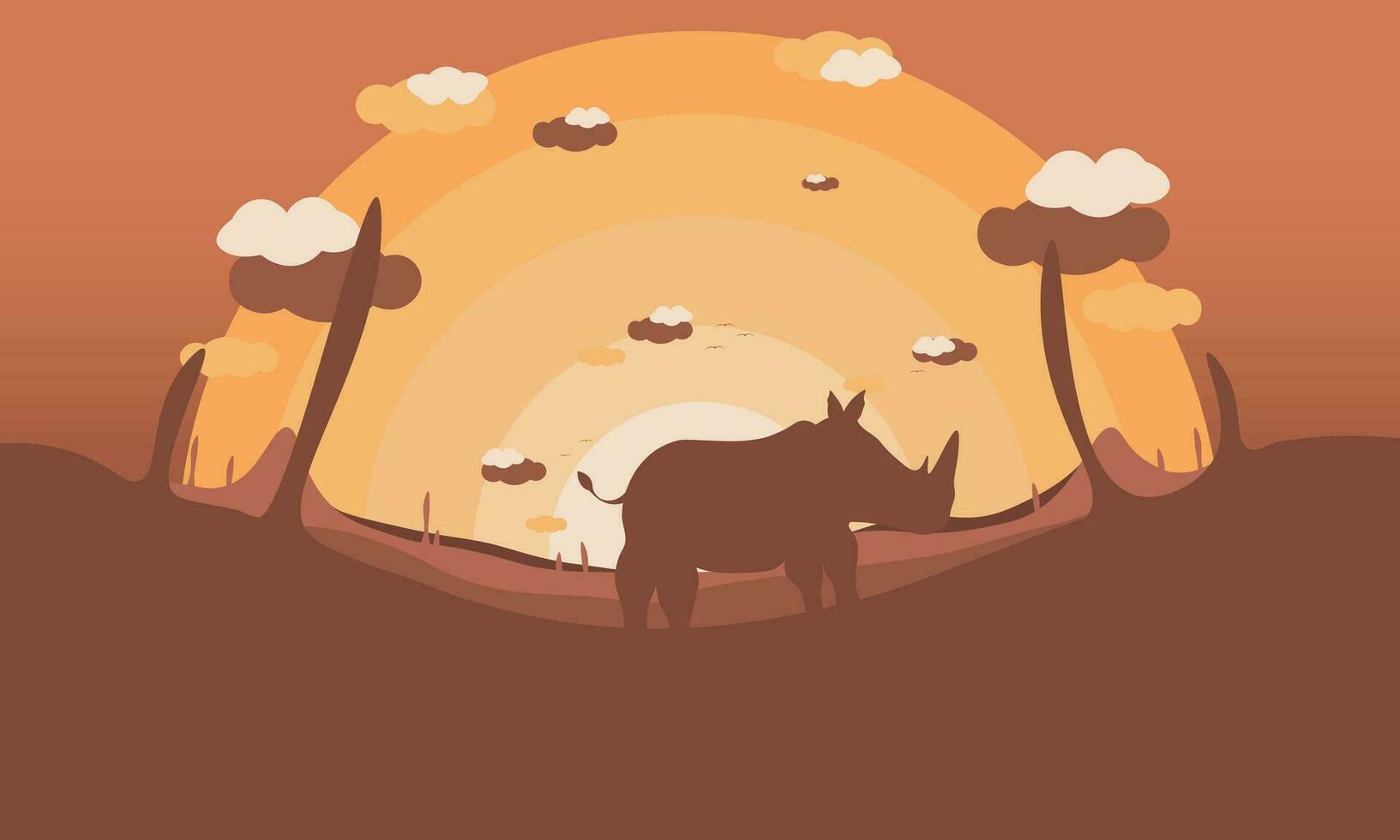This digital artwork, rendered in shades of brown, orange, and red, depicts a stylized rhino silhouette standing on a subtly curved ground, facing right. The rhino, positioned centrally, is devoid of intricate details, showcasing its distinctive horn and small tail in a simple, shadow-like outline. The surrounding environment suggests a desert landscape, with extensions of the reddish-brown ground flanking both sides of the rhino. In the background, a striking semicircular sun or rainbow dominates the red sky, embellished with concentric rings transitioning from dark yellow to white at the core. This celestial feature is accompanied by sparse, multicolored clouds in white, dark brown, and light brown hues. Scattered cacti further enhance the arid, dawn setting of the composition.